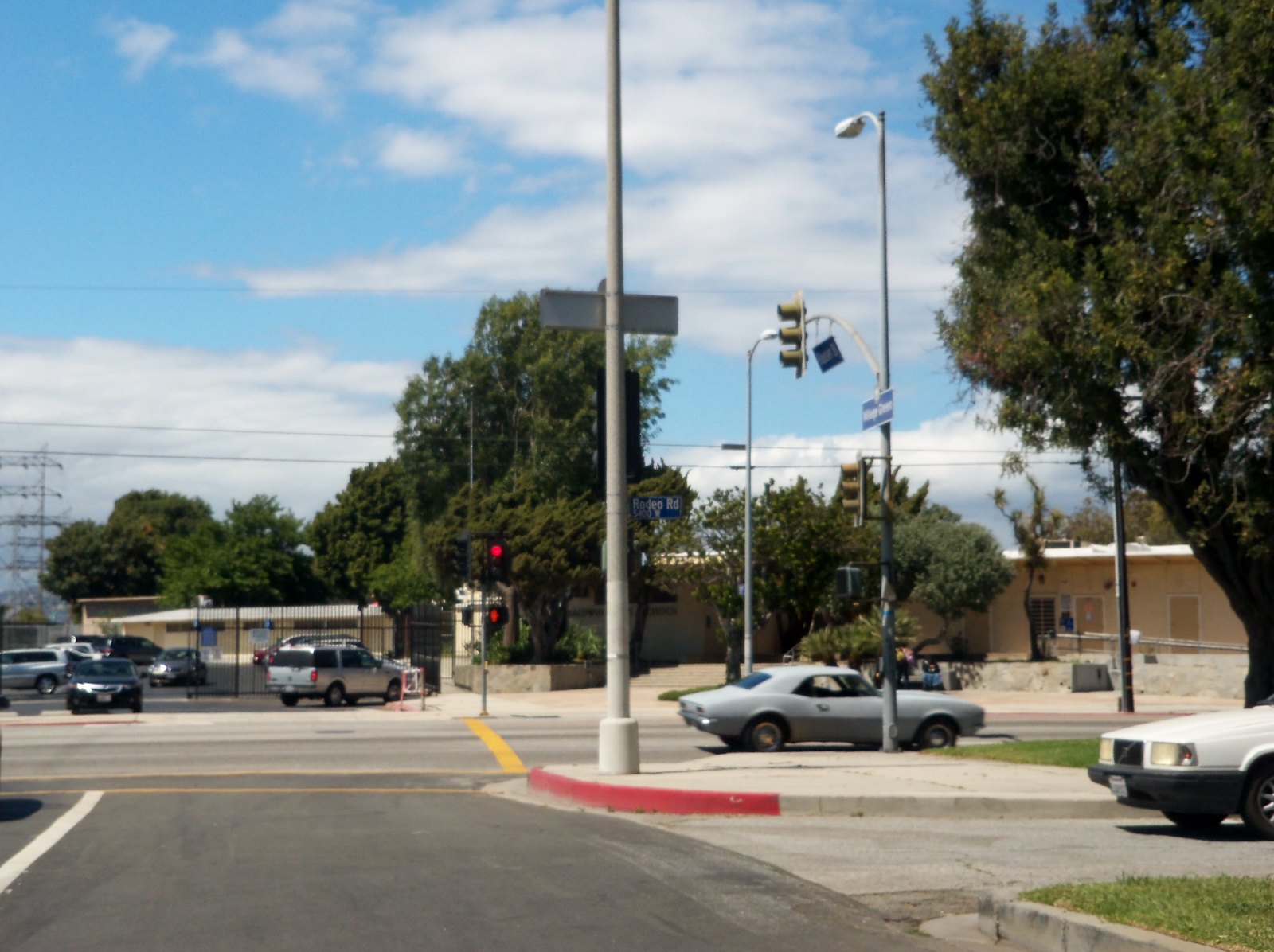The photograph captures a typical suburban-urban street scene, viewed from inside a car positioned on the right-hand side of the road. Just ahead, a driveway branches off from the right, while the engine of a white car encroaches into the image from the same side. The street is characterized by an exceptionally wide sidewalk and a red curbed area, signaling the approach to a three-point intersection. On the intersecting street, a gray car is moving from left to right, adjacent to the red curb.

In the upper right-hand portion of the frame, a large green tree provides a natural contrast to the constructed environment. Beneath this tree, a brick building with a white roof runs horizontally across the lower part of the scene. Centered in the roadway ahead, slightly to the left, is a parking area enclosed by a high chain-link fence, containing two parked cars—one dark-colored and one gray.

In the background, a low-level yellowish building with a white roof stands before a tree line. The horizon is marked by a tree line, above which thickly settled clouds are scattered across a blue sky, completing the composition of this suburban-urban tableau.